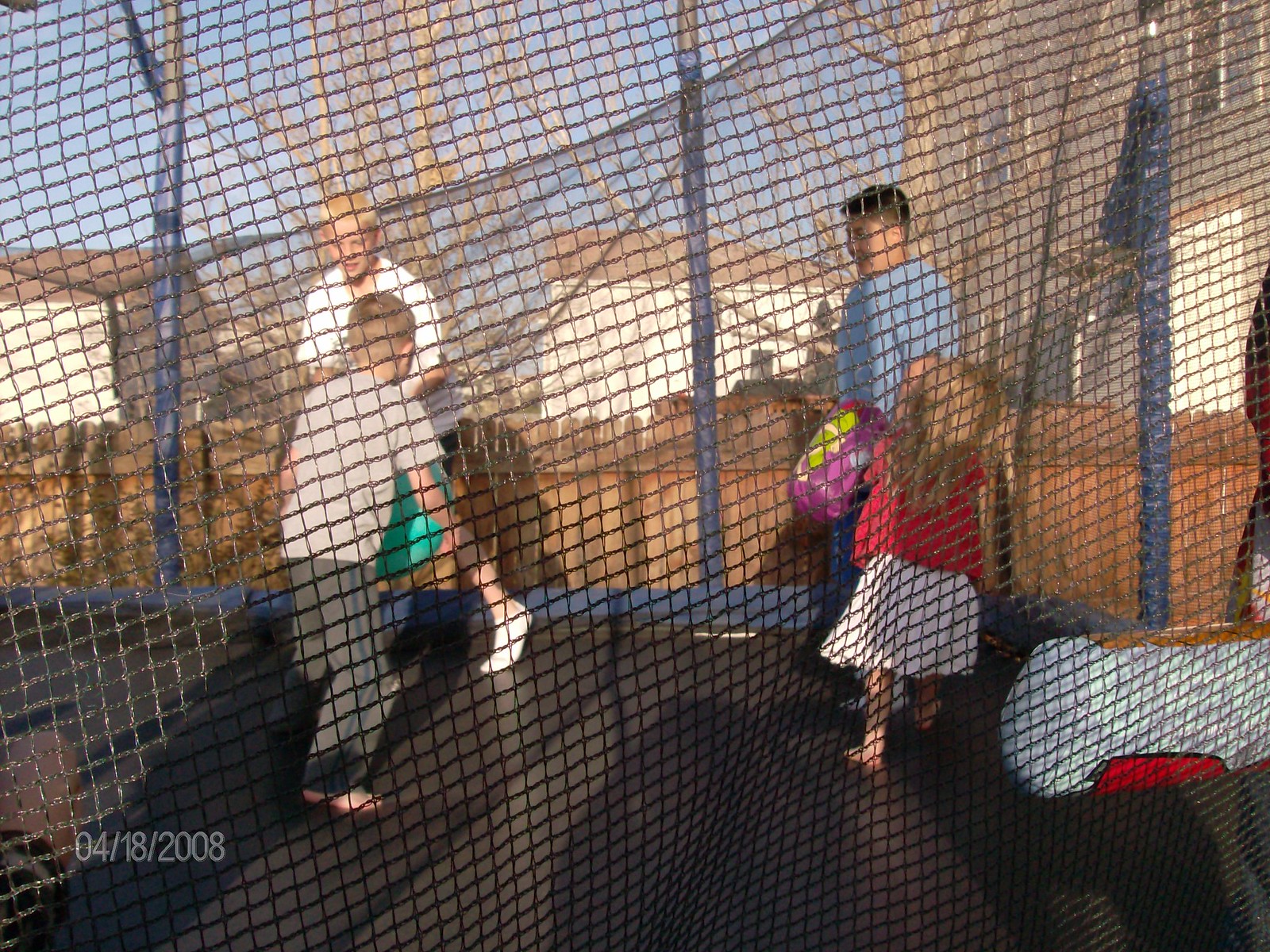The image captures a lively backyard scene of four children on a round trampoline, which includes blue padded poles and black netting for safety. The black trampoline bed is the center of their play, and none of the kids are jumping at the moment; they seem to be engaged in playing with inflatable soccer boppers. The timestamp on the bottom left corner of the photo reads "4-18-2008." The youngest is a small girl, estimated to be about three or four years old, dressed in a red shirt and white skirt. The boys appear to be a bit older: one is around six years old, wearing gray pants and a tan t-shirt with blond hair. Another boy, possibly around eight or nine, is in a blue shirt with dark hair, and the oldest, who might be a teenager, is a blond-haired boy in a white shirt. The backdrop features residential houses, reinforcing the domestic and familial atmosphere of this warm-weather day.